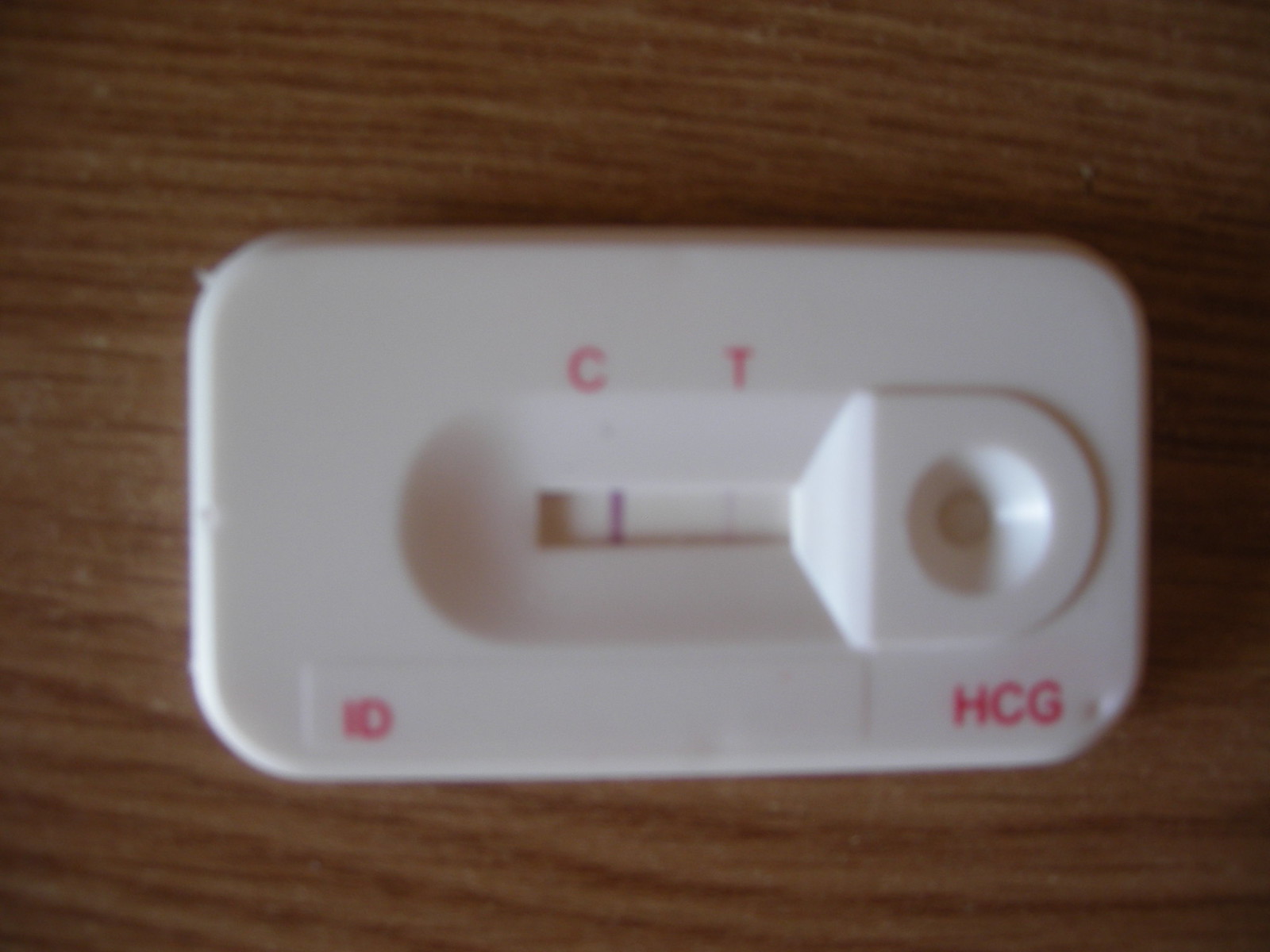This image features a home test kit that is either a COVID test or a similar diagnostic tool. The test kit is rectangular with softly curved edges and predominantly white in color. On the bottom-left corner of the kit, there are some identification letters, while the bottom-right corner prominently displays the letters "HCG" in red uppercase font.

In the center of the kit, there is an oval-shaped window with a clearly visible vertical indicator line inside. Directly above this oval window, the letters "C" and "T" are marked, indicating control and test lines respectively. Beneath these letters, a thicker line is visible under "C" and a thinner line is present under "T."

To the right of the oval window, there is a small depressed area resembling a cone with a central pad, which is likely the spot where a sample is to be deposited onto the test kit.

The kit itself is placed on a surface that could either be wooden or a simulated wood plastic material, featuring a green and tan color scheme.